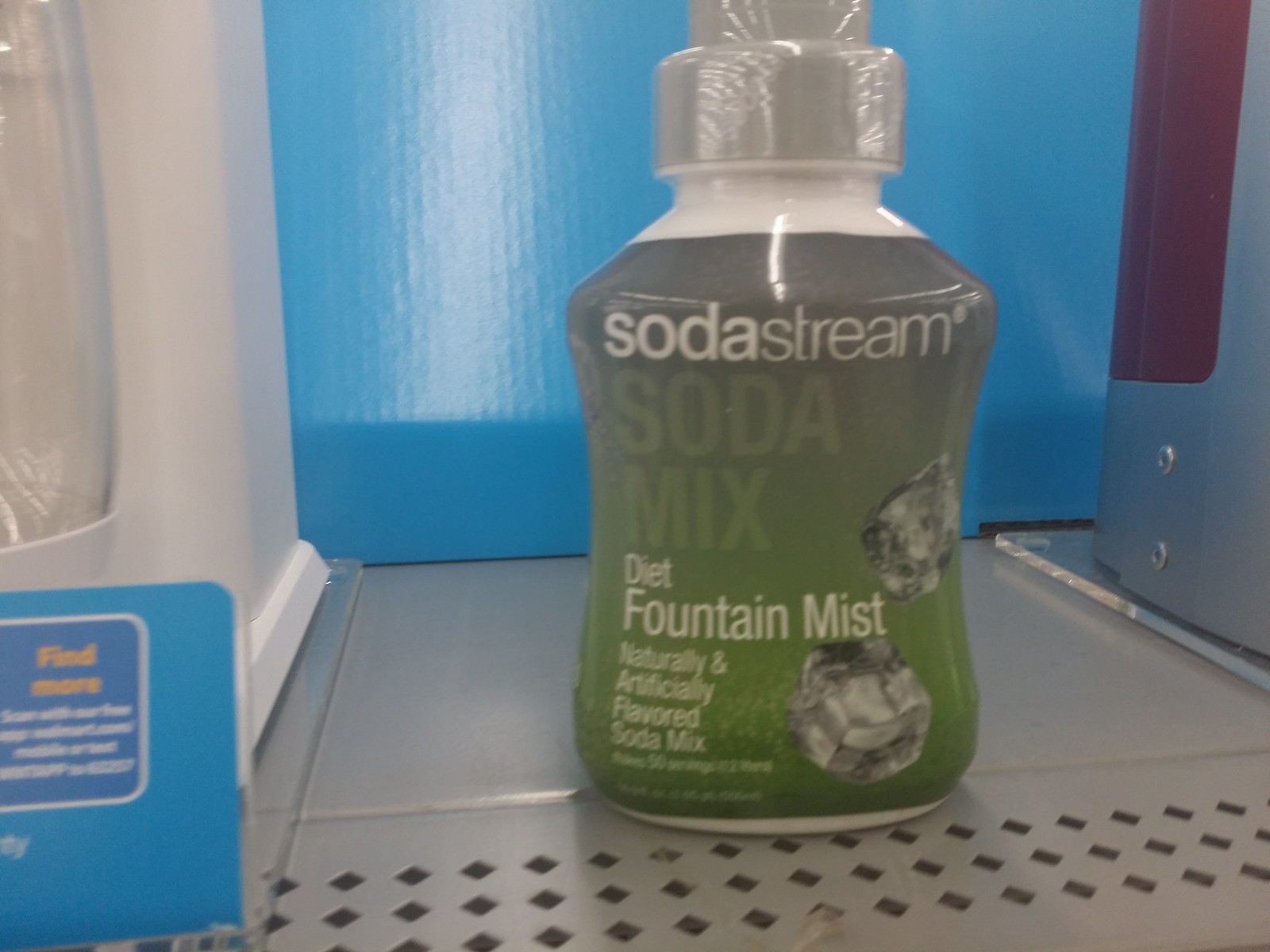An up-close photograph captures a green plastic bottle of SodaStream SodaMix, labeled Diet Fountain Mist. The bottle, designed akin to a knockoff of Diet Mountain Dew, sits on a perforated gray metal shelf, securely wrapped in its original cellophane seal. The label, starting just below the bottle's short neck, transitions from gray at the top to forest green at the bottom, predominantly featuring green and white fonts. "SodaStream" is printed in white at the top, followed by "SodaMix" in light green, "Diet" below it, and "Fountain Mist" underneath. Two ice cubes float prominently on the label, emphasizing the cool, refreshing nature of the drink. The background is a mix of aqua blue, red, and silver, with a partially visible Walmart label and an indistinct placard on the left that reads "find more." This setup suggests the bottle is within a store display, casually placed by someone browsing the shelf.